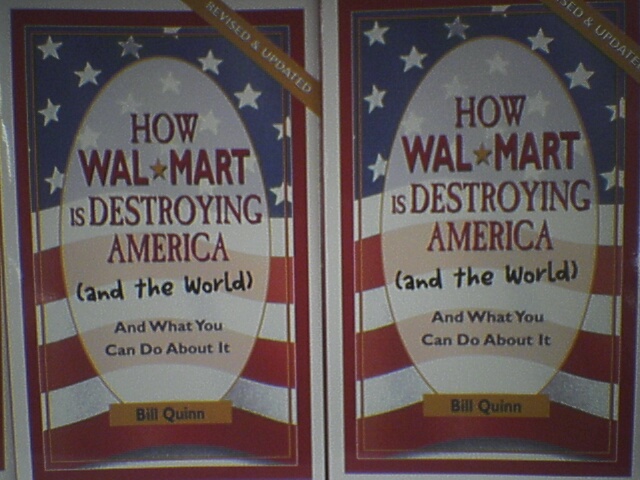The image features two identical side-by-side copies of what appears to be a book cover. Each cover depicts a zoomed-in segment of the American flag, where the top half shows the blue field with white stars, and the bottom half displays the red and white stripes. Dominating the center of the cover is a large, vertically-oriented white oval with a gold trim, through which the flag remains visible. Inside the oval, in bold red letters, is the main title: "How Walmart is Destroying America." Below the title, in a smaller black font within parentheses, it reads "and the world," followed by "and what you can do about it" in black font. A yellow banner along the bottom of the oval bears the author's name, Bill Quinn, in black text. Additionally, in the upper right-hand corner, a gold diagonal banner states "Revised and Updated" in white text. The border of the cover is red, enhancing the patriotic theme.